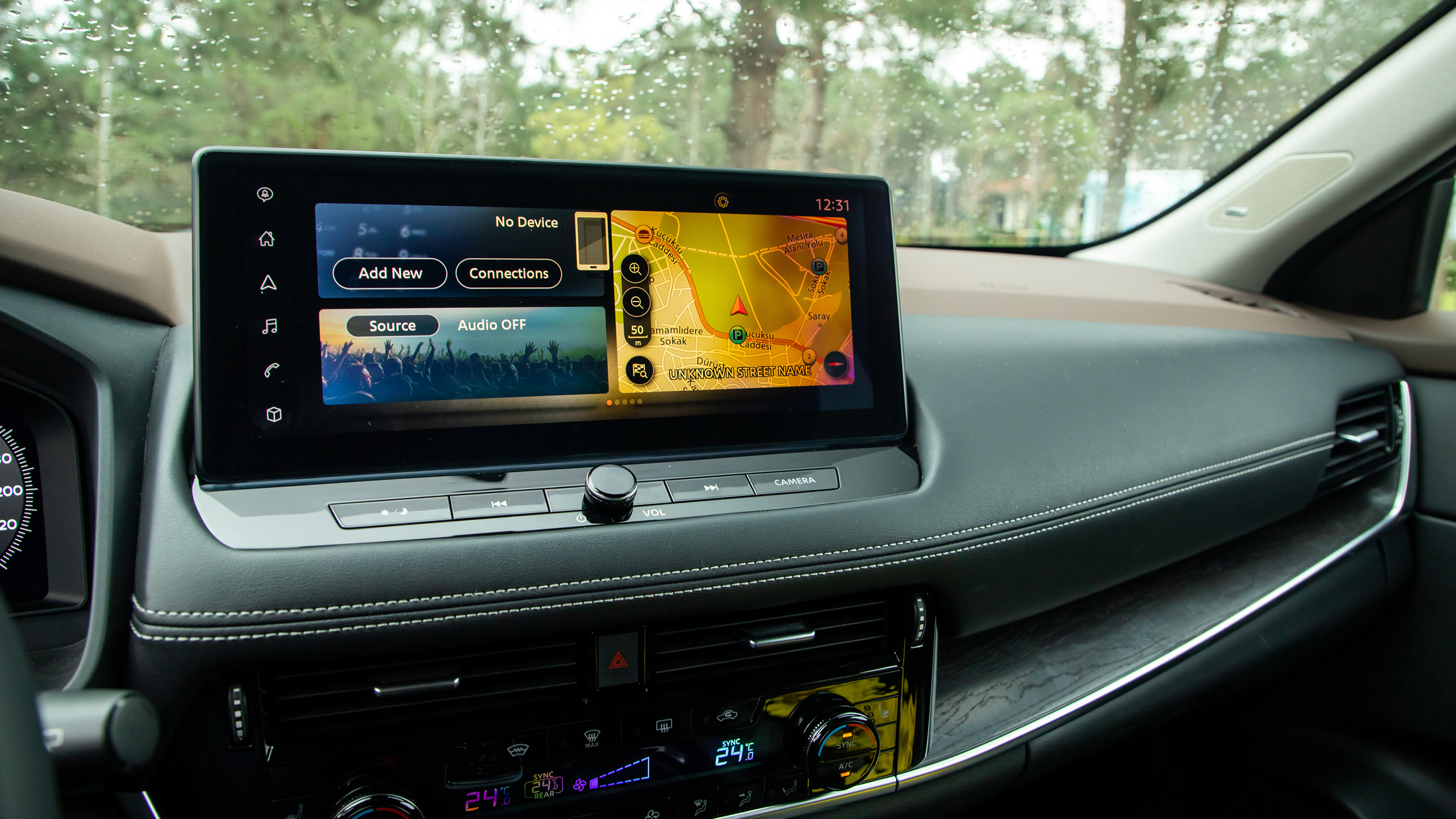This photograph captures the interior of a car from the driver's seat perspective, looking through the windshield on a rainy day. Raindrops are clearly visible on the windshield, with trees and hints of a lake in the background. The focus is the car's central console featuring a sophisticated infotainment system. The console displays a wide, rectangular split-screen interface. The right half of the screen shows a GPS map, while the left half is divided into two sections: one for Bluetooth connections, displaying “No Device,” “Add New,” and “Connections,” and another for audio settings, showing “Source” and “Audio Off.” The screen also displays the time, 12:31. Surrounding the screen are capacitive touch buttons for functions such as home, music, phone, and navigation. Below the screen are additional controls for music, including buttons for volume, fast forward, reverse, and a central knob. The dashboard features a combination of light gray leather with white trim and some wood grain accents. Vents and additional controls, including a dual-zone AC, are situated beneath the infotainment system. Partial elements of the steering wheel, indicator stick, and speedometer are visible at the left edge of the image. The overall interior is well-lit and modern, with a clean and polished appearance.